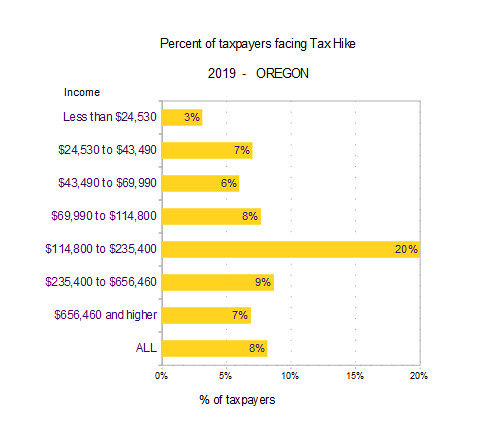This image is a detailed, horizontally displayed bar graph titled "Percent of Taxpayers Facing Tax Hike, 2019, Oregon." The x-axis represents the income categories, which are segmented into roughly $20,000 increments, while the y-axis indicates the corresponding percentages of taxpayers. The graph features bright yellow bars with black and white text.

The income categories and their corresponding percentages are as follows:
- Less than $24,530: 3% (small yellow bar)
- $24,530 to $43,490: 7% (yellow bar)
- $43,490 to $69,990: 6% (yellow bar)
- $69,990 to $114,800: 8% (yellow bar)
- $114,800 to $235,400: 20% (yellow bar)
- $235,400 to $656,460: 9% (yellow bar)
- $656,460 and higher: 7% (yellow bar)
- All income brackets combined: 8% (yellow bar)

The graph clearly highlights that the highest percentage of taxpayers facing a tax hike falls within the $114,800 to $235,400 income range, at 20%, indicating a significant impact on the middle to upper-middle class.